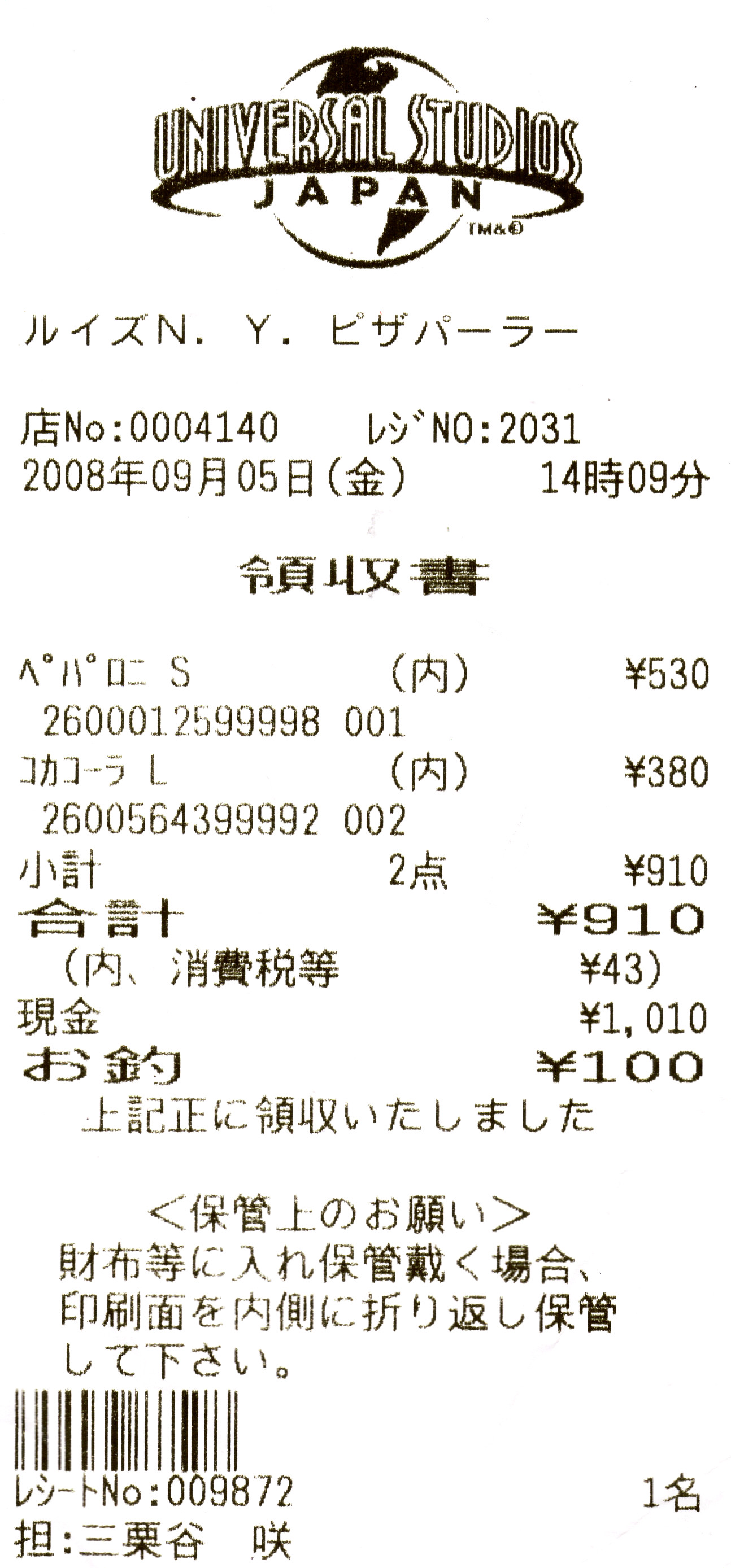The image portrays a tall, narrow receipt from Universal Studios Japan, seamlessly blending into a white background with no visible borders. At the top, the receipt prominently displays the Universal Studios Japan logo, followed by rows of Japanese text. Beneath, a series of itemized entries are accompanied by their respective prices in yen, including amounts such as 530, 380, 910, and 1,010 yen, suggesting multiple purchases. Notably, there is also a barcode positioned in the lower left-hand corner, and alongside it, another string of numbers (009872). The entire receipt is presented in black and white, emphasizing the text and numerical details.